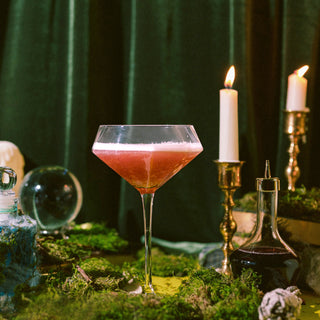The photograph captures an elegant and meticulously arranged setting centered around a single margarita glass, filled with a pinkish-red beverage topped with a hint of white froth. The clear glass sits prominently on a surface that appears to be covered in moss, making it the focal point of the image. Surrounding this central element, the ambiance is accentuated by the glow of thin, white candles, strategically placed in candle holders to the right of the glass. Both candles are alight, casting a warm yellow flame that complements the scene. The backdrop is a dark green curtain, adding a layer of sophistication and depth, hinting at a luxurious, possibly romantic dinner setting. Additional objects include a glass beaker positioned in front of one of the candles and a spherical glass ball to the left of the margarita glass, enhancing the overall composition. The photograph is devoid of any text, allowing the viewer's focus to remain on the elegant display, which is meticulously staged to showcase the appealing appearance of the drink in an indoor setting.